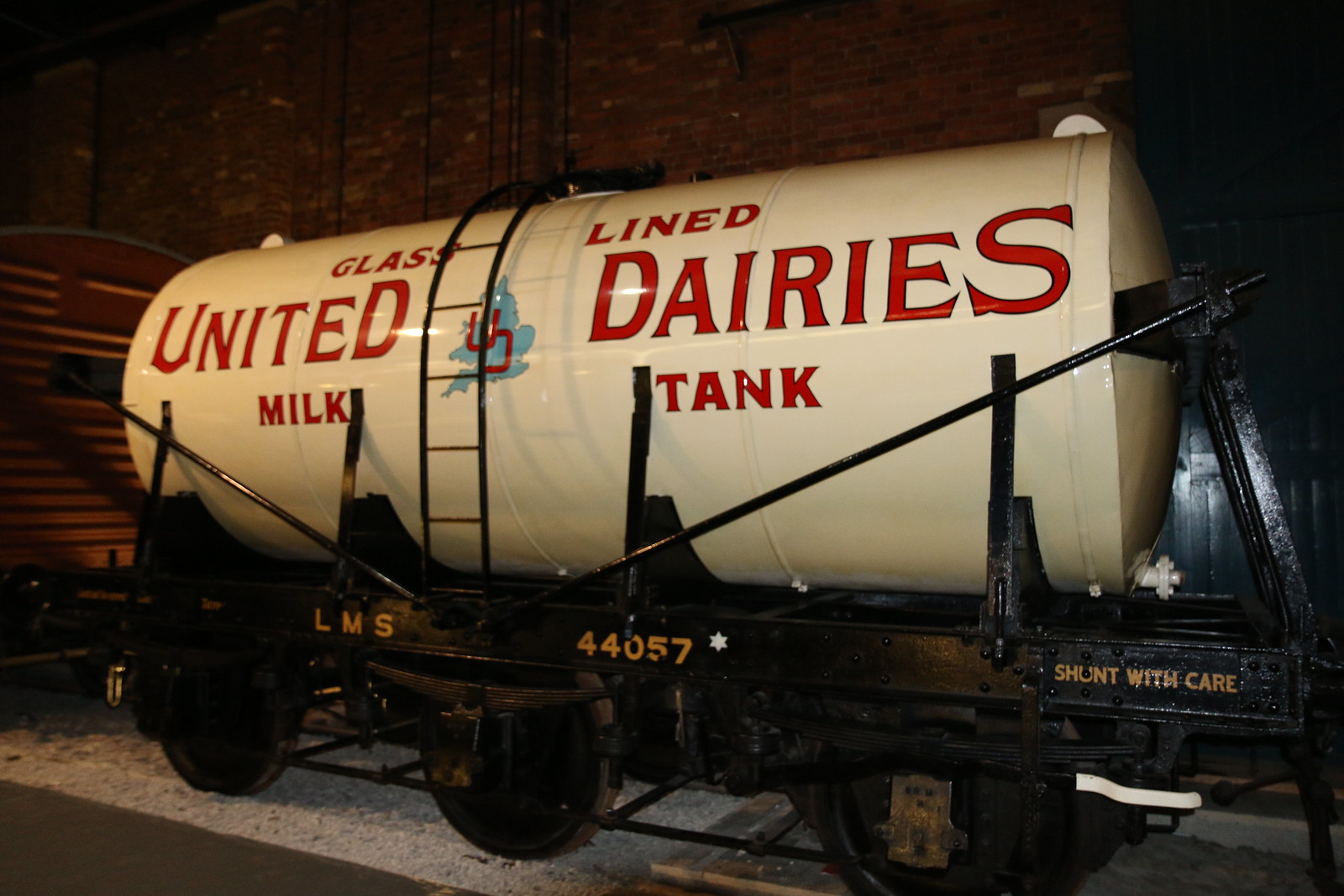The photograph depicts a vintage milk tank mounted on a black six-wheeled railroad car, displayed against a backdrop of a large red brick wall, suggesting the setting is inside a museum. The black rail car, visible from its right side, features gold lettering with "LMS" followed by "44057" and the cautionary phrase "Shunt With Care." Atop the rail car is a prominent white cylindrical tank labeled "Glass Lined United Dairies Milk Tank" in bold, red text. Embedded in the center of this text is a blue image of Great Britain, overlaid by a large red "U.D." logo. A black ladder ascends from the base of the rail car to an inlet or opening at the top of the tank. To the left of the milk tank, a red railroad car, possibly a caboose, can be seen peeking into the frame. The detailed design and preserved condition of the cart and tank highlight the historical significance of the milk transportation system.